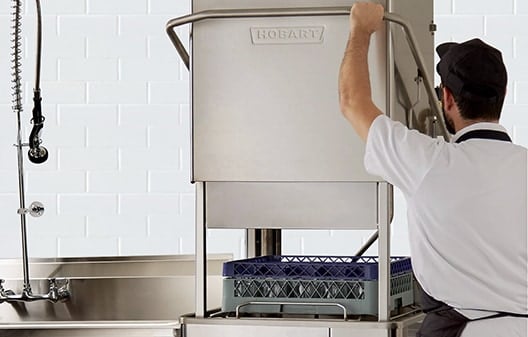In the image, a man is depicted operating an advanced dishwashing machine in a bustling commercial kitchen. The background features distinctive white subway tiles commonly found in professional culinary environments. Situated on the left side of the image is a large stainless steel wash basin, equipped with a prominent and highly functional faucet. This faucet extends upward with a spring-loaded structure that supports a removable wash head, designed for efficient dish cleaning.

To the right, we observe the Hobart automatic dishwasher, a stainless steel apparatus notable for its boxy shape and a handle at the top. This machine is engineered to lower over racks of glass drinkware, providing thorough cleaning and sterilization. The man, donned in a crisp white short-sleeved shirt, a black apron, and a matching black ball cap, appears focused as he operates the dishwasher. He is seen preparing to pull the handle down to engage the machine, with two plastic crates of glassware ready for the wash cycle. His attire also includes a dark beard, further highlighting his professional yet practical appearance in this fast-paced kitchen setting.